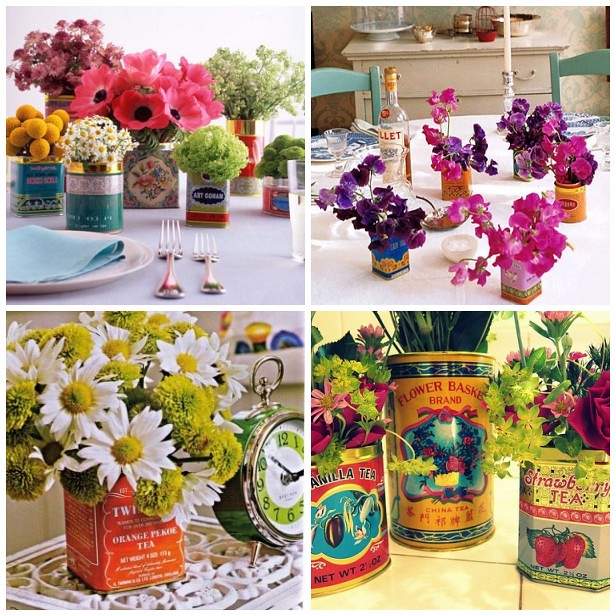The composite image features four distinct photographs, each showcasing creative floral arrangements using repurposed tin canisters. In the top left corner, a white plate with a folded blue napkin and two silver forks are placed against a backdrop of various tin canisters filled with vibrant flowers, including white blooms with yellow centers, pink flowers, and small yellow flowers resembling cotton balls. Moving to the top right image, a round white table is set with blue wooden chairs, a large white candle, and a bottle of wine. Several tea canisters repurposed as vases hold pink and purple flowers, adding a dynamic touch to the setting. 

The bottom left photograph features a red can labeled "Twining's Orange Pico Tea," brimming with white-petaled flowers with green centers, surrounded by greenish-yellow flowers. An old-fashioned green alarm clock is positioned beside the can on a tiled white wooden surface. Finally, the bottom right image showcases three tea canisters labeled "Vanilla Tea" in red with gold trim, "Flower Basket Brand China Tea," and "Strawberry Tea," each overflowing with an array of colorful flowers. The compositions across these four photographs display a harmonious blend of colors and creatively use everyday containers for floral arrangements.